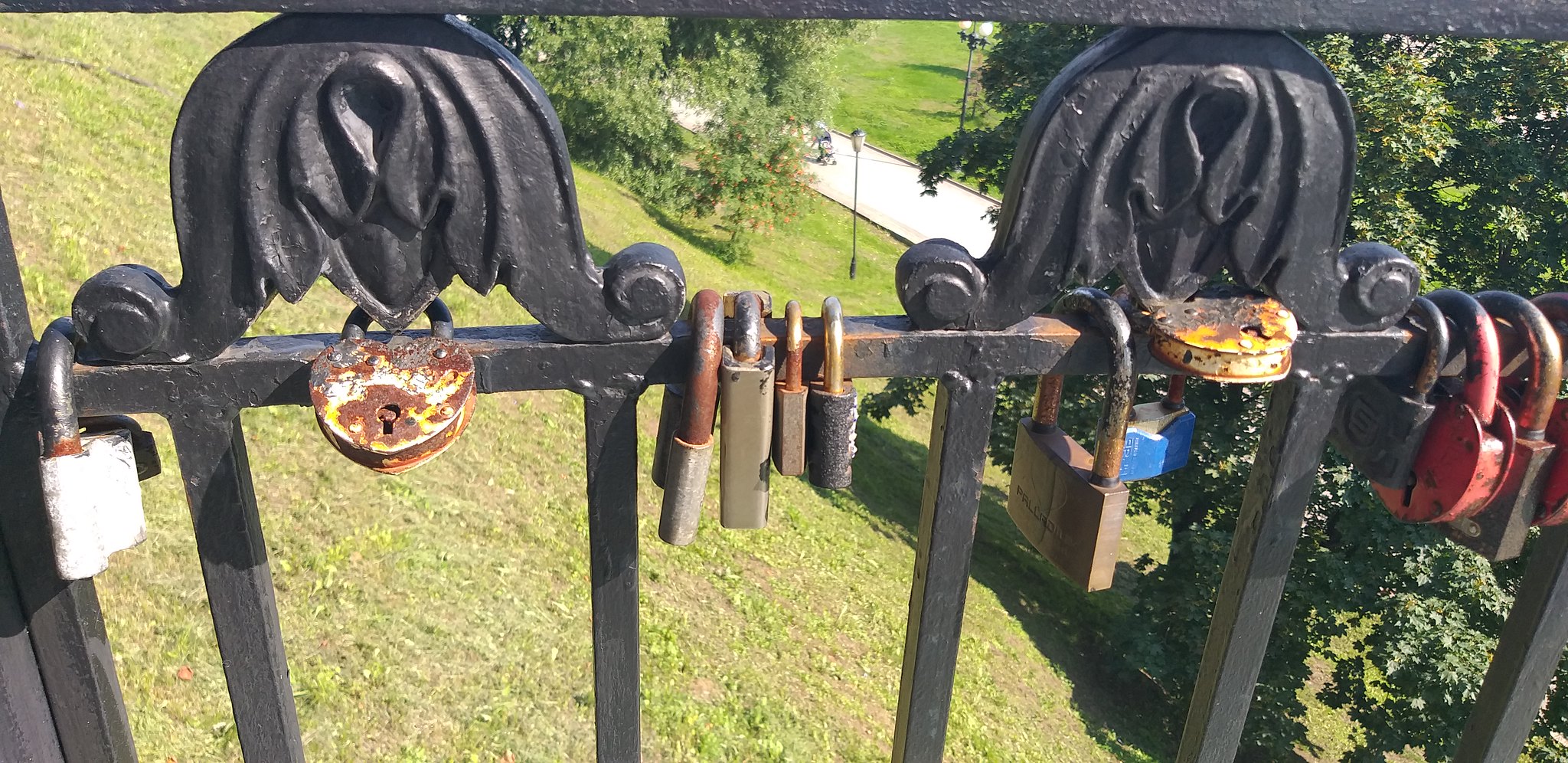The image captures a close-up landscape view of the top portion of a black wrought iron gate adorned with multiple padlocks of varying shapes, sizes, and colors, including heart-shaped and square ones. The locks, all showing signs of age and rust, are attached to the top horizontal bar of the gate. Distinct padlocks with chipped white, yellow, and blue paint, as well as a notably rusted red one, stand out among the collection. The gate features decorative metal adornments resembling inverted U-shapes or stylized angel wings positioned on either side of the top bar. Beyond the gate, a sloped hill with lush green grass and scattered trees descends to a road lined with streetlights and a distant sidewalk, where a person is seen pushing a trolley.